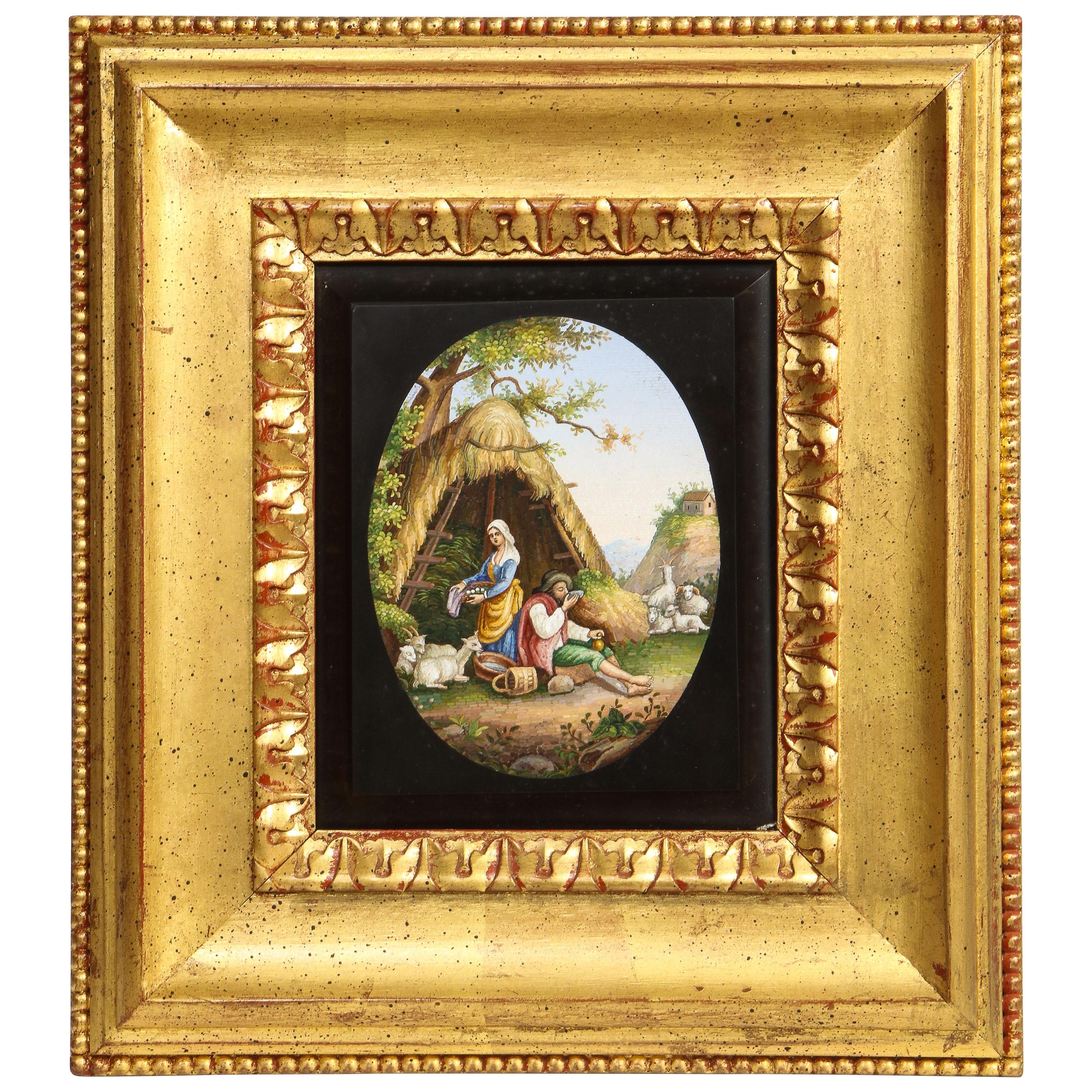This image showcases a detailed oil painting with a pastoral biblical theme, framed in an exceptionally ornate gold frame. The central scene depicts a man draped in a cloak, taking a rest and drinking from a cup. Behind him stands a woman who appears to be tending to a flock of sheep, further enriching the rural atmosphere. They are situated in front of a quaint A-frame house with a thatched roof, protected by the leafy branches of a sizeable overarching tree. In the background, a tranquil hill with a small house perched atop is visible, accompanied by more sheep grazing. The painting itself is oval-shaped, encased in a black matting with an oval cutout, and it is surrounded by a striking wide, textured, and bronze-colored frame adorned with intricate patterns and a touch of red patina. This frame significantly amplifies the presence of the small, yet evocative, piece of art within it.